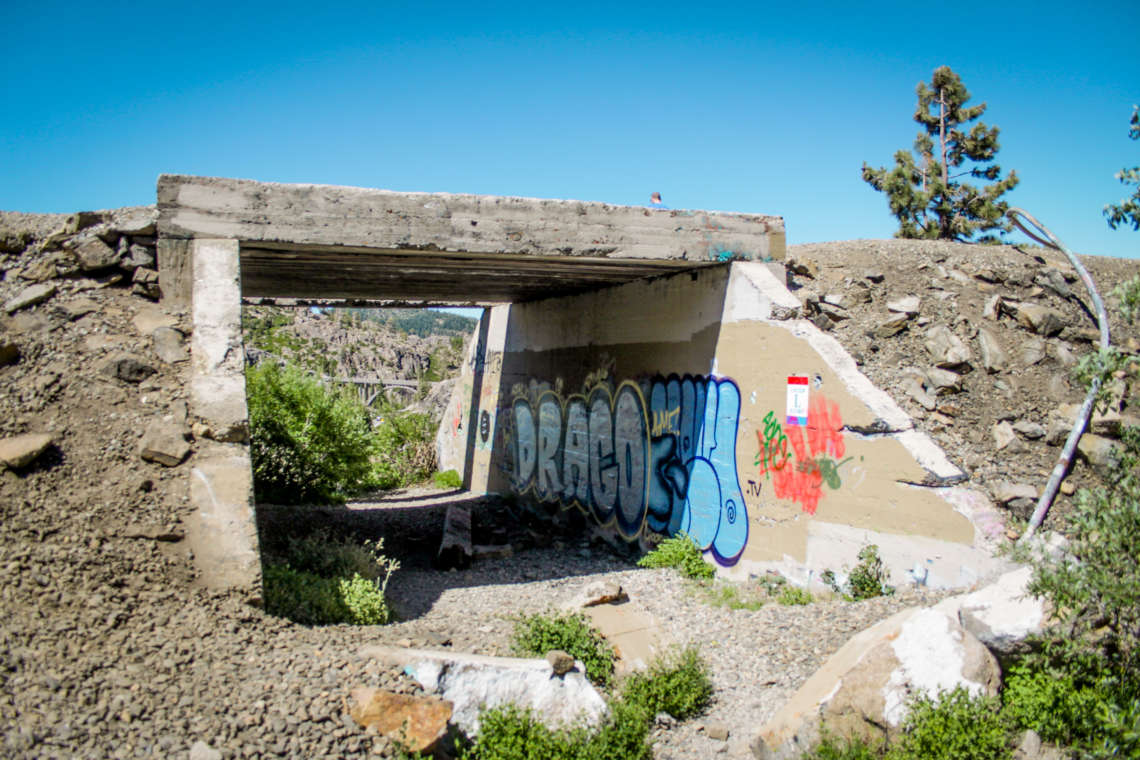The image depicts an abandoned and desolate cement underpass, surrounded by a natural outdoor environment. The scene shows a small tunnel-like structure, once used as an underpass, now filled with rocks, gravel, and sand. Rock formations and soil line the area around the entrance, which is partially blocked by stone. Vegetation, including a notably shriveled plant, grows in the vicinity, with some leaves visible at the top right corner and just beyond the tunnel. Inside the tunnel, a mural with the word "Drago" painted in blue can be seen among other indistinguishable letters and colorful graffiti in red and green. The defunct structure, with its retaining wall heavily marked by graffiti, evokes a sense of abandonment amidst the encroaching natural elements.